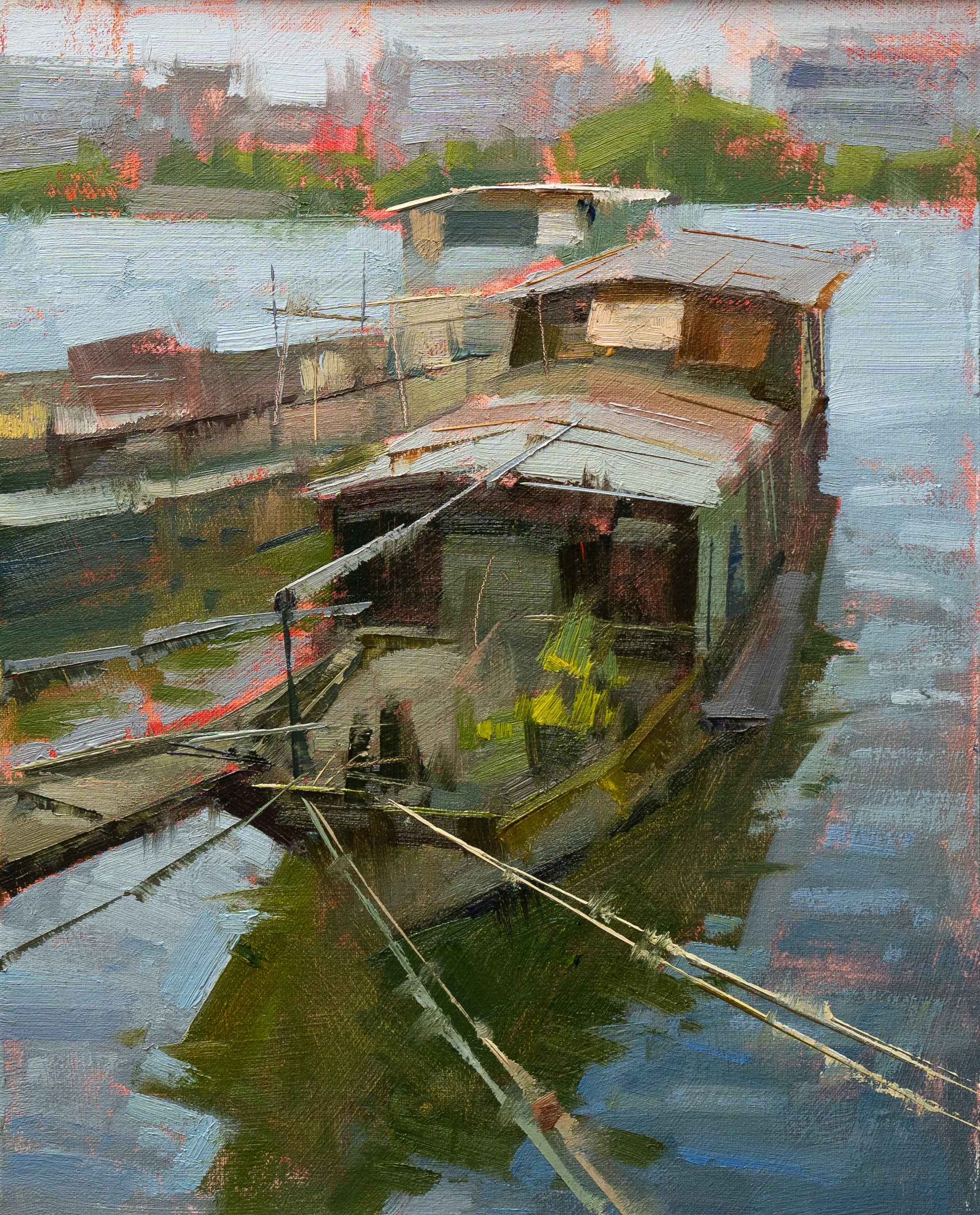The painting depicts a serene scene along a winding river, reminiscent of the tranquil waterways of Vietnam. Central to the composition is a boat navigating the river, tethered by what appears to be ropes or wires to either the shore or adjacent boats. This connectivity underscores the communal and functional aspects of river life, where boats often serve as both homes and workplaces for the inhabitants, reflecting the traditional lifestyle of the region. The painting employs a realistic palette with muted, earthy tones that capture the somewhat murky, dark waters of the river, enhancing its naturalistic portrayal. Though the strokes are somewhat blurred, adding a soft, almost impressionistic quality to the scene, the details remain discernible, effectively conveying the essence of life along these storied waters.